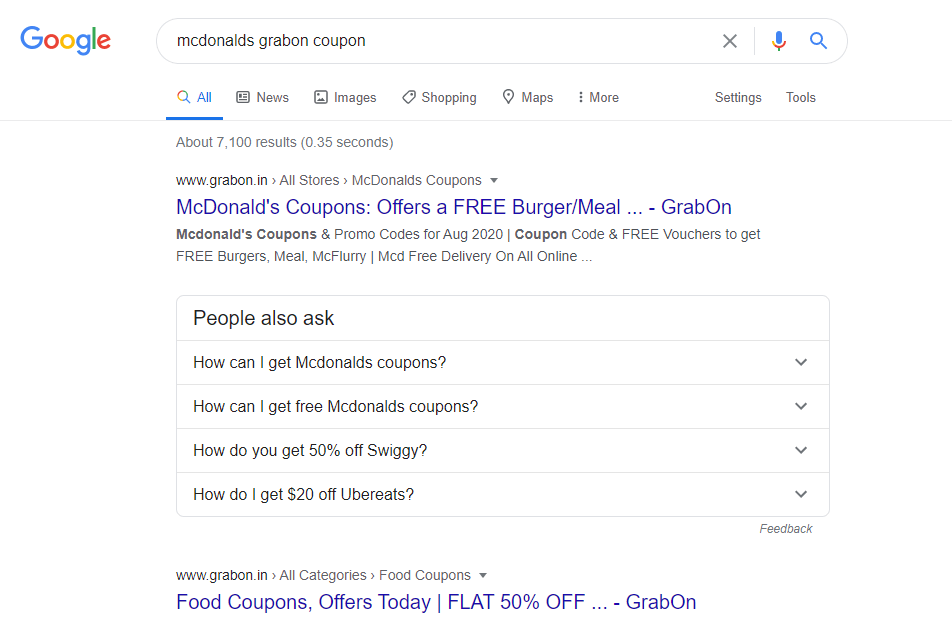The image depicts a screenshot of a Google web search results page. At the top, the colorful Google logo is prominently displayed, signaling the search engine used. The search query entered is "McDonald's Grab on coupon."

Beneath the search bar, the standard Google navigation tabs are visible, including "All," "News," "Images," "Shopping," "Maps," as well as a drop-down option labeled "More." At the far end, there are the "Settings" and "Tools" buttons. The search results indicate there are a total of 7,100 results, fetched in 0.35 seconds.

The primary search result heading reads "McDonald's coupons offers a free burger meal grab on." Below this, there is a section titled "People also ask," which lists relevant questions such as "How can I get McDonald's coupons?", "How can I get free McDonald's coupons?", "How do you get 50% off Swiggy?", and "How do you get $20 off Uber Eats?"

At the bottom of the screenshot, there is a link to www.grabon.in, which offers food coupons and deals, featuring a promotion for today's offers with a flat 50% off on Grab On.